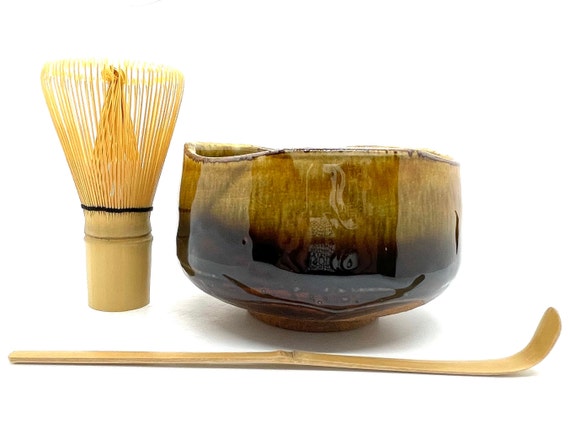The image showcases a brown glazed ceramic container with distinct features. The lower portion of the container is a deep, dark brown color, while the upper section presents subtle golden hues. Positioned on the left side of the container is a cluster of yellow reeds, seemingly nestled in a wooden holder. In the foreground, a wooden stick is prominently displayed. The stick, resembling a hockey stick with its slightly upward-curved end, could potentially double as a massage stick. The detailed textures and colors in the image highlight the craftsmanship of the ceramic container and the natural elements surrounding it.